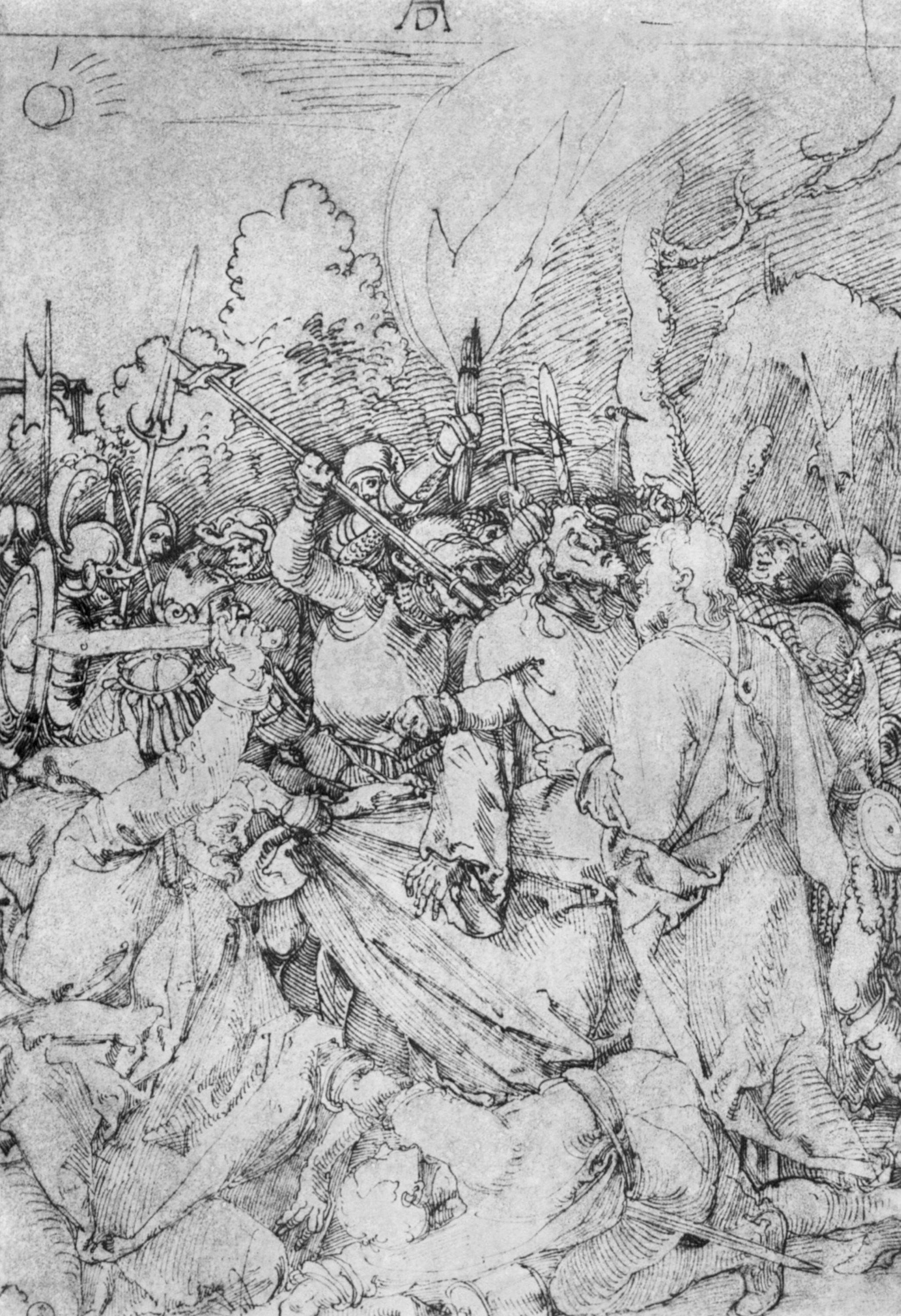The black-and-white sketch depicts a tense and dramatic scene reminiscent of ancient Roman or medieval times. Central to the image is a solitary man with white hair and flowing robes, standing resolutely at the center, facing a throng of armed aggressors. The attackers, positioned predominantly on the left side of the drawing, brandish a variety of weapons including spears, swords, and pitchforks, and appear poised to strike. On the right side, individuals either confront the attackers or lie on the ground, seemingly subdued or injured. The scene exudes a sense of impending violence or recently concluded conflict. Adding to the dramatic atmosphere, a sketch of the sun is situated in the upper left corner, suggesting the event unfolds in daylight, while an outline of trees in the background frames the chaotic tableau. The monochromatic shades of gray, white, and black enhance the stark and gritty feel of this detailed pencil illustration.